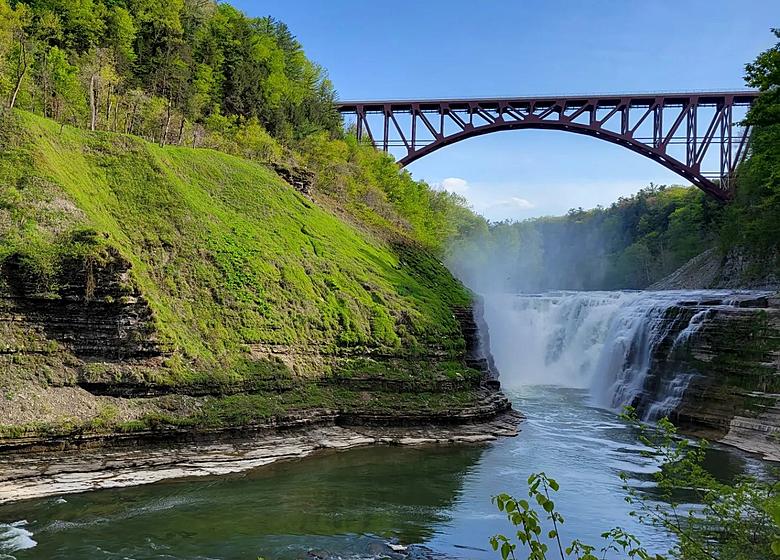In this vibrant color photograph, an arch-shaped metal bridge spans the upper third of the image, positioned above a series of cascading waterfalls. The bridge, brown and picturesque, connects a hillside dotted with trees on the left to a rocky, grassy area on the right. The waterfalls, originating from nearly the top of the image, tumble over flat plateaus of rock before converging into a small canyon, lined with green moss on its rocky face. This canyon directs the flowing water toward the foreground, eventually feeding into a broader body of water. The entire scene is set against a backdrop of blue sky and scattered white clouds, providing a vivid and scenic tableau.